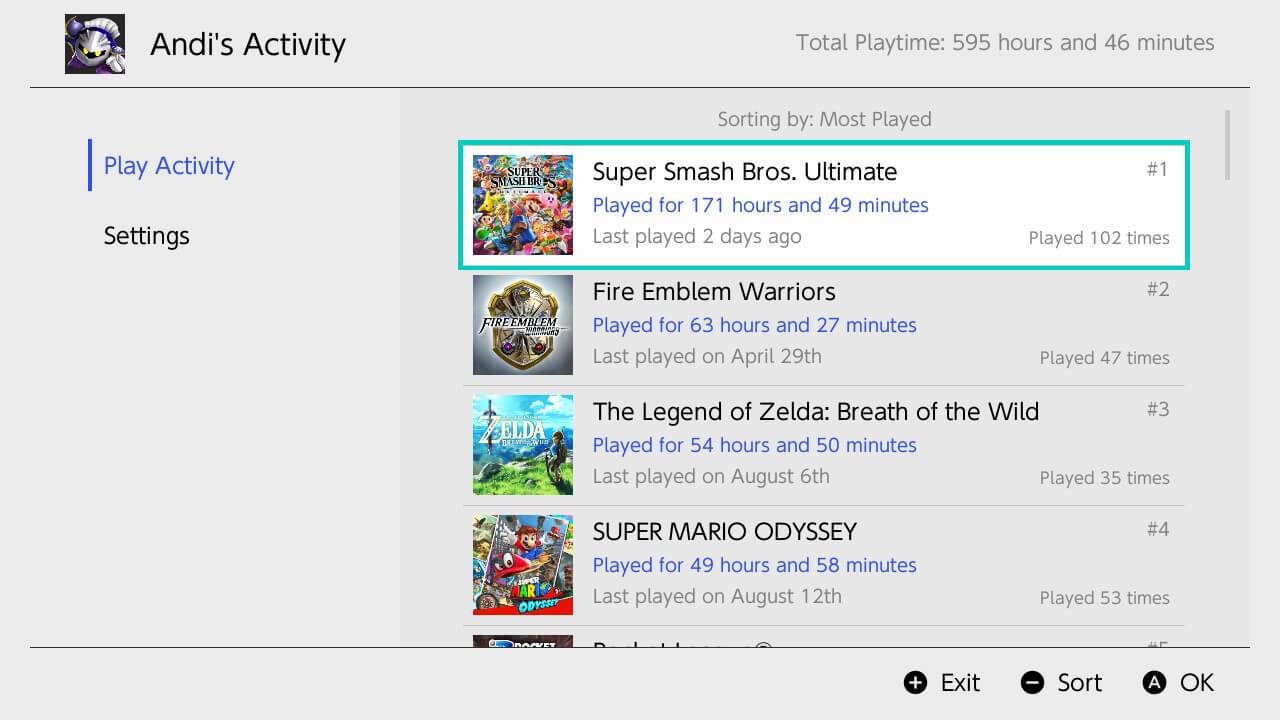The image showcases a horizontally-oriented rectangular interface displaying Andy's gaming activity. The upper left section of the image features a grey background with the text "Andy's Activity" in black. Positioned on the right side of this section, text indicates "Total Play Time: 595 hours and 46 minutes." Directly below, a grey horizontal line separates the header from the rest of the content.

On the left side, two tabs are visible: "Play Activity," which is highlighted in blue with a corresponding blue line, and "Settings," which remains in black. Centered in the middle of the interface, it indicates that the content is "Sorted by Most Played."

Beneath the sorting information, there are four list items, though the fourth one is partially cut off and not fully visible. Each item is contained within a white rectangle bordered by a distinct color associated with the respective game.

1. The first item is highlighted with a turquoise border and lists "Super Smash Bros. Ultimate," showing a total playtime of 171 hours and 49 minutes. This game, marked as number one, was last played two days ago and has been played 102 times.
   
2. The second item details "Fire Emblem Warriors," played for 63 hours and 27 minutes, last played on April 29th. This game is numbered two and has been played 47 times.
   
3. The third item features "The Legend of Zelda: Breath of the Wild," with a total playtime of 54 hours and 50 minutes. This game was last played on August 6th, is listed as number three, and has been played between 33 and 35 times.

4. The fourth item displays partial information for "Super Mario Odyssey," showing a total playtime of 49 hours, although further details are cut off from the view.